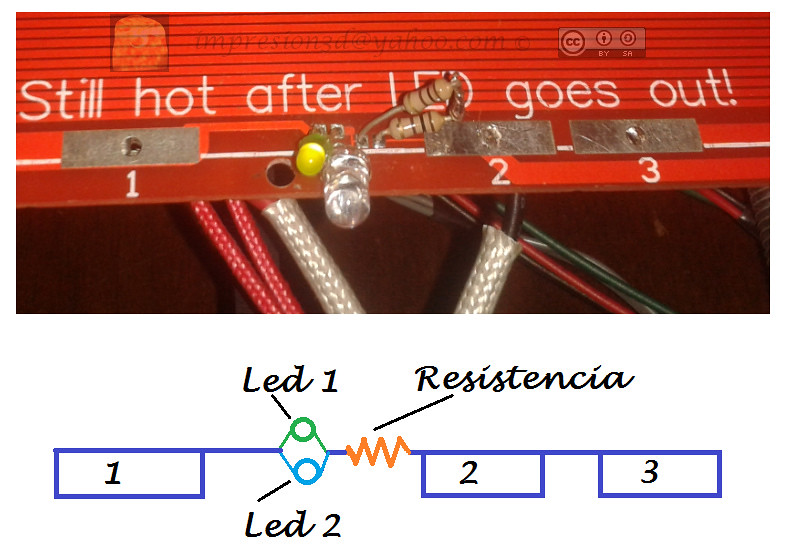The image depicts a detailed close-up of a red circuit board used for electrical maintenance, featuring prominently an LED light and a power transistor. In white text at the top left, it warns, "Still hot after LED goes out!" Exclamation point. Surrounding the board are various wires: red, white, silver, black, and a combination of green and red. Below the circuit board is a digital drawing that explains the wiring connections. It includes three columns labeled 1, 2, and 3, illustrating how the wires and components are interconnected. The diagram also labels sections as LED 1, LED 2, and Resistance. You can also see a faint website URL "Impressioned at Yahoo.com" with a copyright symbol, along with symbols depicting closed captioning (CC) and other icons.